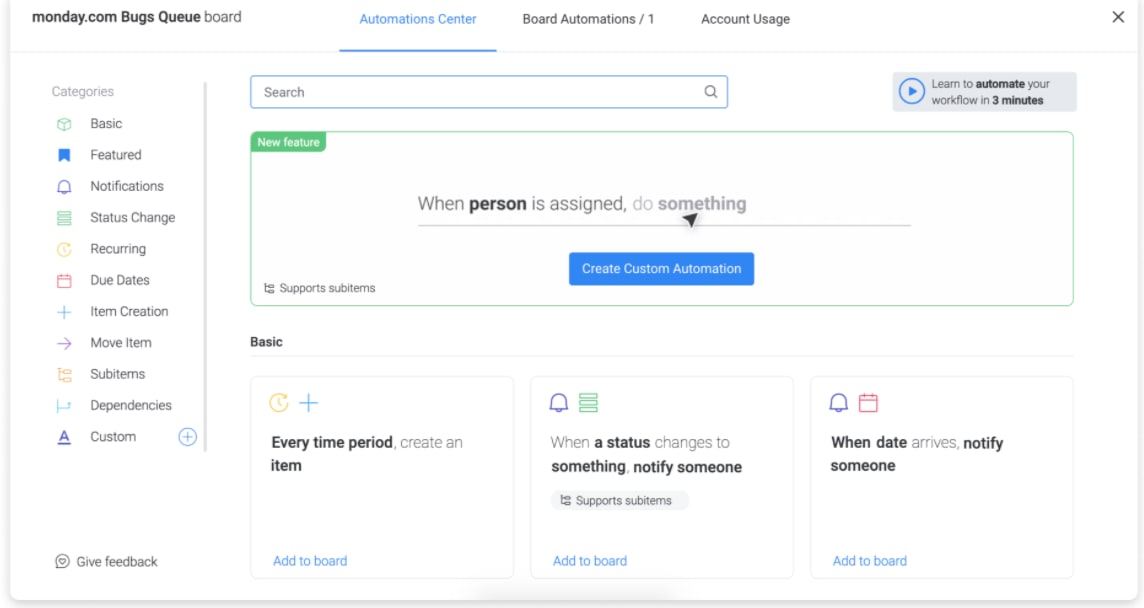The image appears to be a screenshot of a computer interface displaying the monday.com platform, specifically focusing on its automation features. The background is plain white, ensuring that all on-screen elements are clearly visible.

At the top left corner, the screen has a label reading "monday.com bugs keyboard." Across the top, there are three main navigation options: "Automation Center," "Board Automations," and "Account Usage." The "Automation Center" tab is highlighted in blue and underlined, indicating the user is currently on this section.

To the right of these options is a search bar with the prompt "Learn to automate your workflow in three minutes," accompanied by a play button, suggesting a tutorial video is available.

On the left side of the interface, there's a vertical rectangular menu labeled "Categories," listing various automation categories: basic, featured, notifications, status change, recurring, due dates, item creation, move item, sub-items, dependencies, and custom.

The center of the image features a prominent rectangular section. In the upper left corner of this section, there's a label announcing a "New Feature," followed by a guide starting with "When a person is assigned to do something." Beneath this guide is a large blue button labeled "Create Custom Automation," inviting users to set up their own automation rules.

At the bottom of the screen, three boxes are displayed horizontally. The first box contains a plus sign and the text "Every time period, create an item." The second box has an icon resembling a bell and the text "When a status changes to something, notify someone." The third box features a bell with a calendar icon and the text "When date arrives, notify someone."

The overall layout is clean and intuitive, guiding the user towards setting up various automation rules and exploring new features efficiently within the monday.com platform.